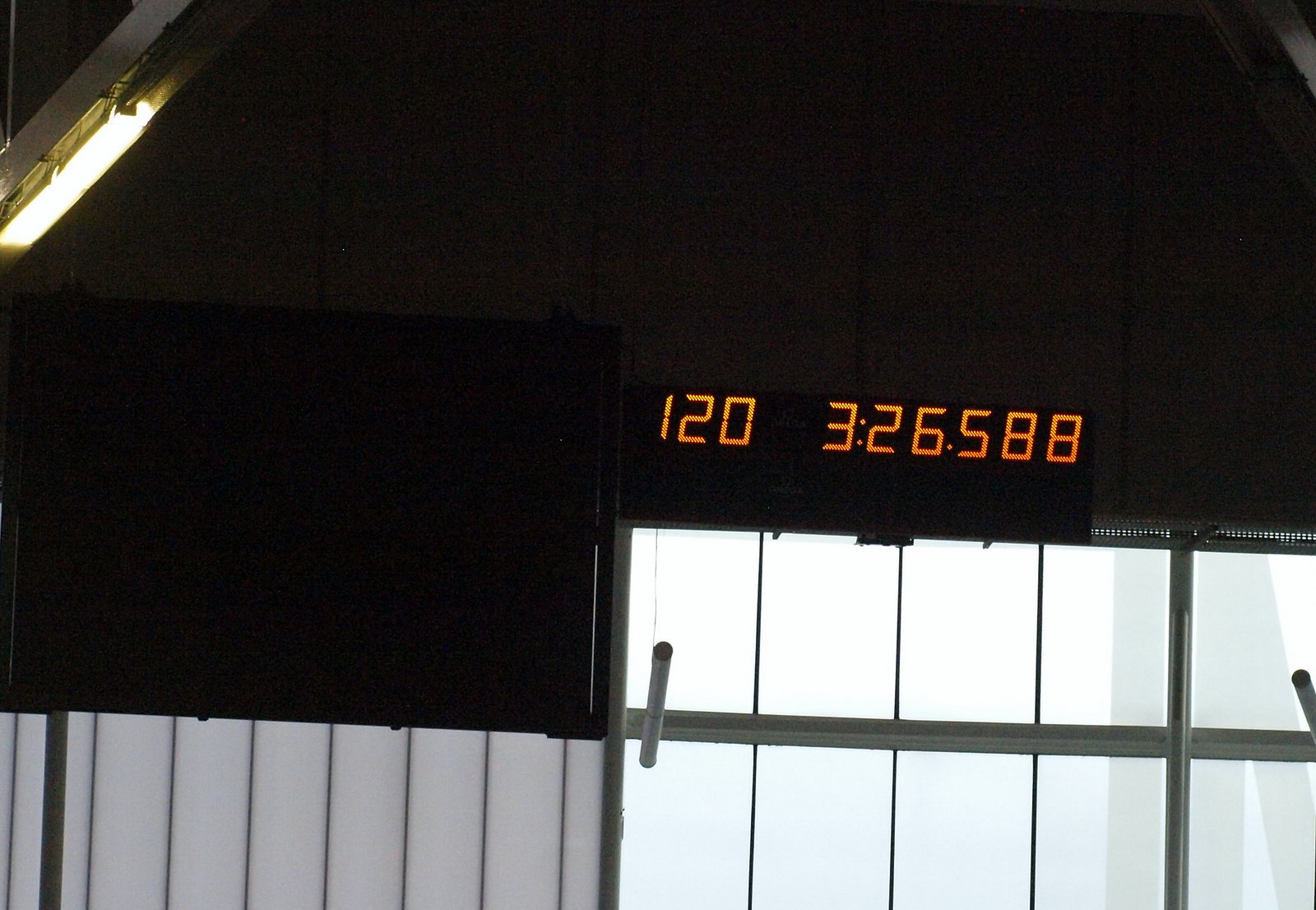The photograph depicts an indoor setting with a stark black background. In the upper left corner, there is a light source that subtly illuminates part of the scene. The primary focus of the image is a large rectangular window stretching from the lower left to the lower right corner, segmented into multiple vertical panes. Above this window, in bright orange-yellow letters, is a numerical display reading "120 326 588," which likely resembles a time-keeping device. Positioned centrally and to the right within the frame, a bar or pipe protrudes from the window area. Additionally, on the left side near the time display, there is a TV mounted on the wall. Shadows, including one tall and thin, reminiscent of the shape of the Washington Monument, can be seen cast against the wall, adding depth and mystery to the indoor scene. The entire photograph maintains a rectangular format, emphasizing the details within its borders.